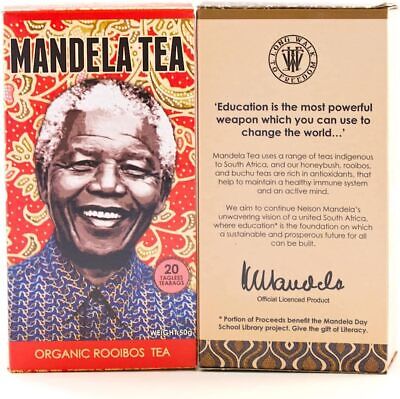This small square image, which appears to be an advertisement for Mandela Tea, features a split design resembling a box, displaying both the front and back. The left side showcases a photograph of Nelson Mandela from the shoulders up, smiling and wearing a blue button-down shirt adorned with white squiggly lines. The background behind him is a vibrant red decorated with white dots and hand-drawn yellow floral patterns. At the top in black letters, it reads "Mandela Tea," while a red stripe at the bottom in white letters proclaims "Organic Rooibos Tea."

On the right side, which represents the back of the box, the background is a light tan color. Prominently at the top, a quote in bold black text states, "Education is the most powerful weapon which you can use to change the world." Below this quote are two small paragraphs of text likely describing the product, accompanied by a signature at the bottom in black ink, and marked as an "official licensed product." The design also includes a stamp-like logo, adding to its official and authentic appearance.